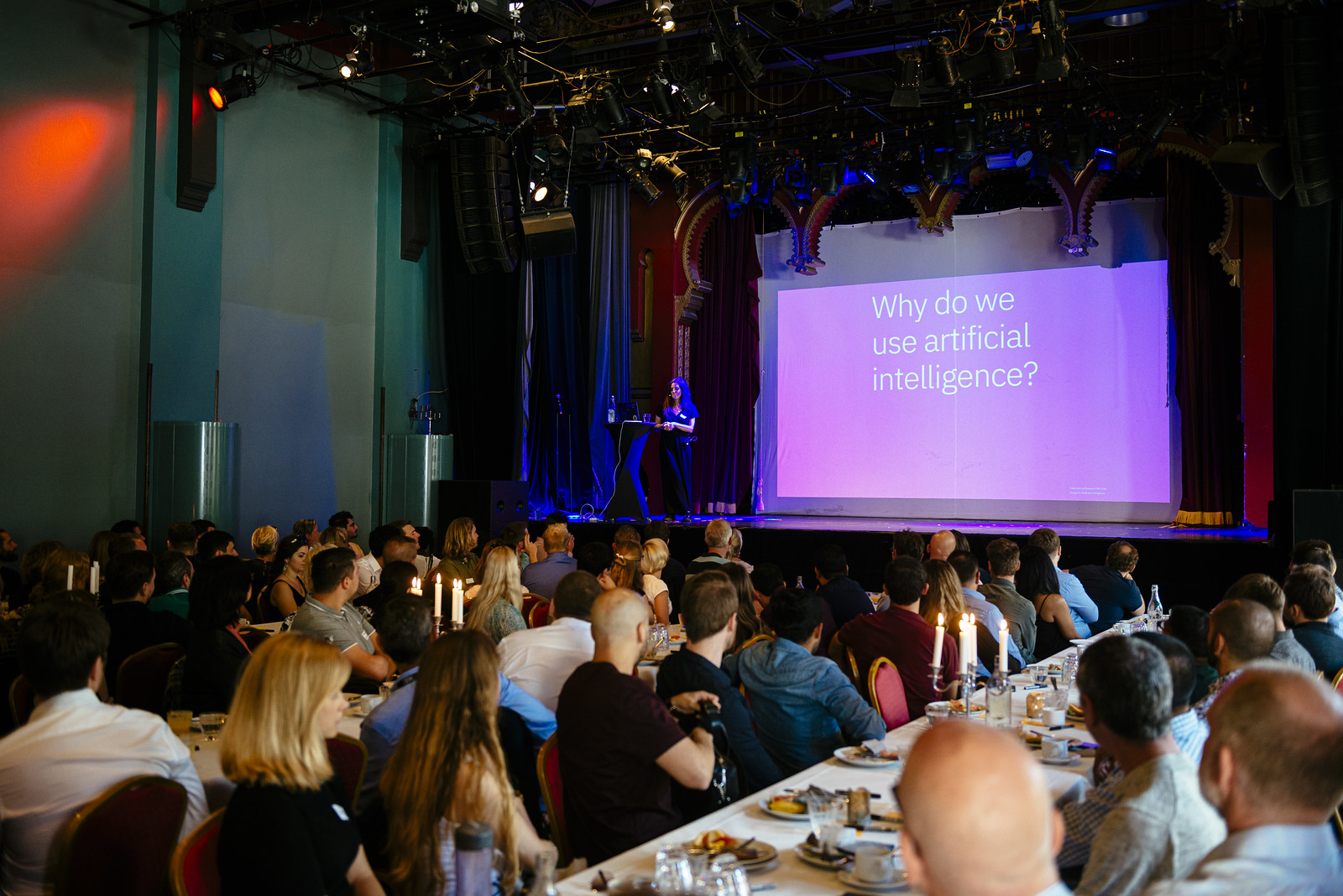The image captures a wide, rectangular scene of a dimly lit venue where a large audience is seated at long banquet tables adorned with dishes, cups, and food, engaging in a formal event. The bottom half of the image shows the guests facing a stage located in the top right, where a petite woman in a dark outfit stands at a centrally positioned dark podium. She is illuminated by blue light, contributing to the muted ambiance. Behind her, a massive projection screen displays a purple slide with white text that reads, "Why do we use artificial intelligence?" The upper portion of the image reveals multiple lighting rigs and spotlights suspended from the ceiling, while on the left side, green walls and short pillars add to the ornate setting, reminiscent of a space designed for theatrical performances. The overall scene suggests a focused and somewhat young audience, intensively engaged in the presentation.